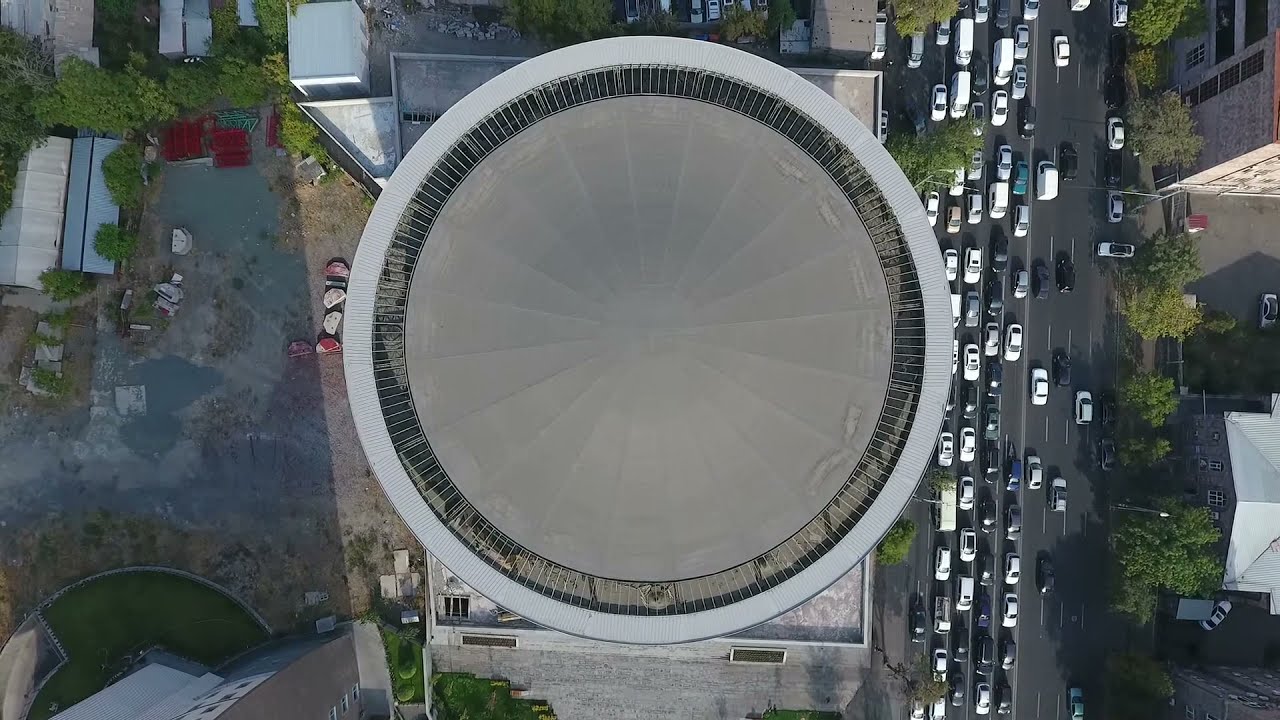The aerial view image captures an urban landscape featuring a variety of structures and natural elements. The centerpiece of the image is a roof centered in the middle, colored in shades of gray. To the right of this main building, there is a busy street lined with a mix of black, white, and blue cars. The street is accompanied by dashed white lines, indicating many lanes and frequent traffic flow. On the left side of the image, there's an overgrown area resembling a storage yard, dotted with shed-type buildings that have white and blue roofs, surrounded by green trees. Additional structures are noted including a circular building with a gray boundary, a beige center, and brown railings. Scattered throughout the left and bottom sections are buildings with varied roof colors—blue, beige, silver, and white, situated among trees. Despite the mix of urban and natural elements, no text is visible within the image.